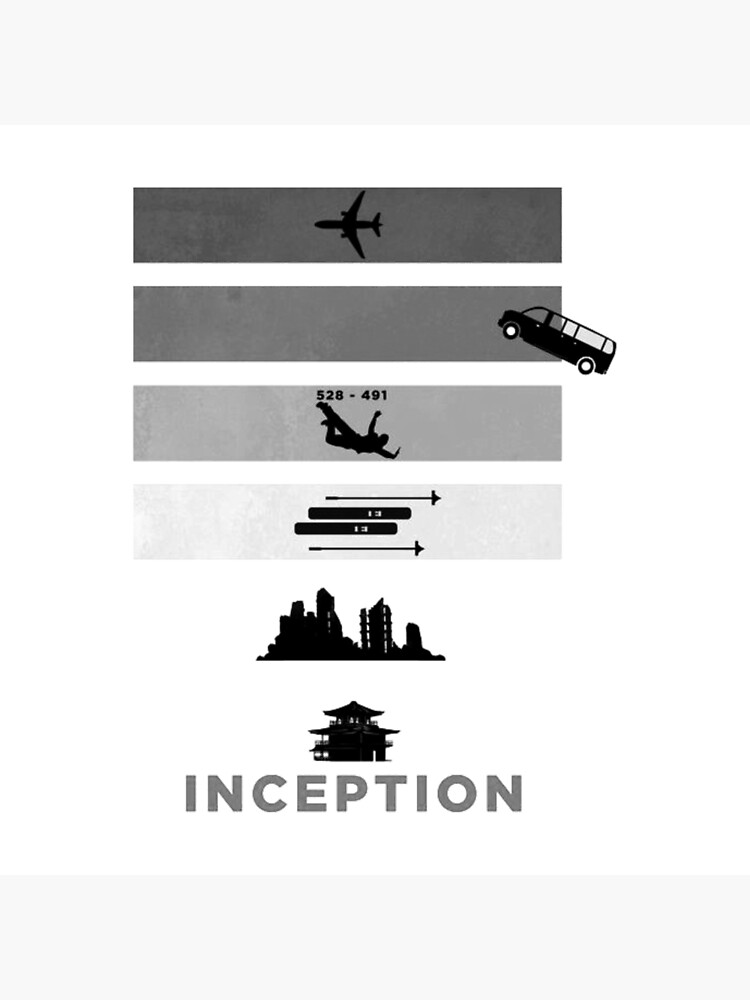The vertically-arranged movie poster for "Inception" features six horizontal bands of varying shades of gray. At the top, a charcoal banner showcases a dark black silhouette of a passenger airplane flying to the left. Below this, a slightly lighter charcoal banner depicts a cargo van precariously tipping off the right edge. In the third, lighter gray band, a person in a black design outfit is seen free-falling with the numbers "528-491" above them. The fourth lighter gray banner includes a central section with two lines and the number "13," flanked by upward and downward arrows, and an additional arrow pointing to the right side of the poster. Below that, a silhouette of a cityscape is visible, leading to the final band which presents a stylized image of a traditional Japanese pagoda. The word "Inception" is prominently placed at the bottom of the poster, in a medium shade of gray.